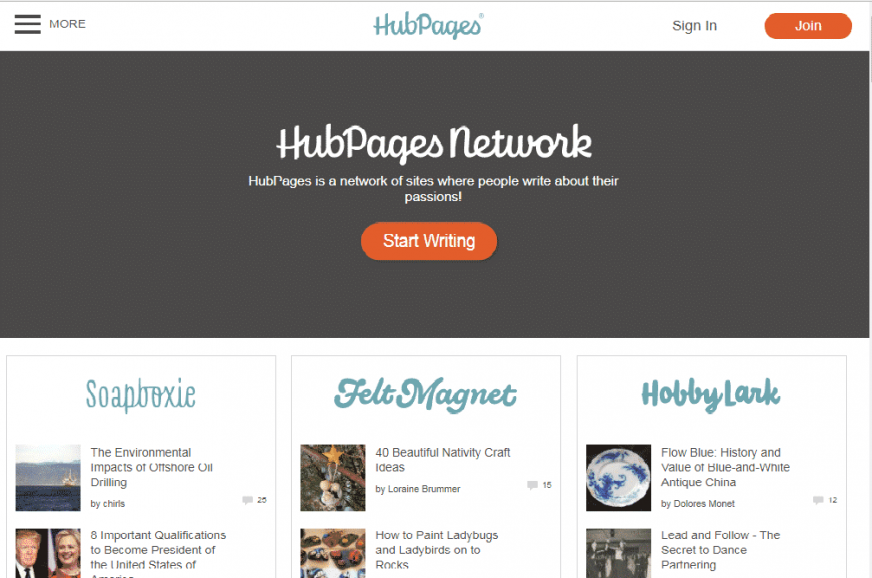The image depicts a partial web page layout for HubPages. Starting from the top left, there is a white border featuring a three-line "hamburger" menu icon, followed by the word "More." Centered at the top is the HubPages logo. On the right side are a "Sign In" option and an orange "Join" button.

Directly beneath, there is a dark grey box occupying about half of the page's width, with the text "HubPages Network" displayed in white. Below this, a tagline reads, "HubPages is a network of sites where people write about their passions." An orange "Start Writing" button is prominently placed beneath the tagline.

The page is divided into three main sections featuring different niche sites:

1. **Soapboxy**:
   - An article titled "The Environmental Impacts of Offshore Oil Drilling" by Chris, accompanied by an image of a waterway with an offshore drill.
   - Below is a photograph of Trump and Hillary Clinton with the headline, "Eight Important Qualifications to Become President of the United States of America."

2. **FeltMagnet**:
   - This section highlights an article titled "Forty Beautiful Nativity Craft Ideas" by Lorraine Brummer, illustrated with an image of felt craft items.
   - Another article in this section is "How to Paint Ladybugs," featuring images of ladybugs painted on rocks.

3. **HobbyLark**:
   - Displays an article titled "Flow Blue: History and Value of Blue and White Antique China," accompanied by an image resembling the Earth from space, later identified as a blue and white antique plate.
   - Another article is "Lead and Follow: The Secret to Dance Partnering," though the accompanying black-and-white image is indistinct.

The detailed descriptions and categorized sections provide an organized and comprehensive visual guide to the various topics featured on HubPages.